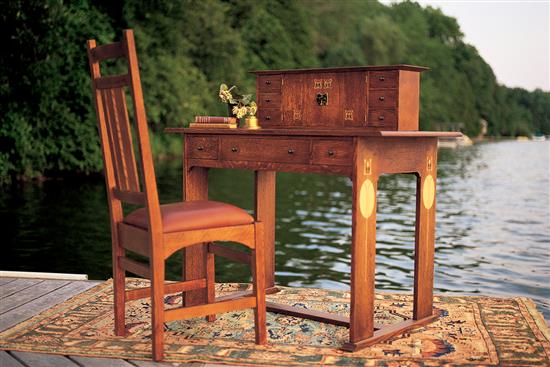The photograph captures an unusual and captivating scene during the daytime: a wooden antique desk and matching chair placed on a Persian-style rug on a dock by a tranquil lake. The ornate rug features light brown, yellowish, and orange hues, adding warmth to the setting. This antique desk, boasting a small cabinet with three doors on each side attached to its surface, also has a set of three drawers along the front and wide, elegantly decorated legs with oval accents. On the desk, there's a charming flower arrangement and a couple of books, enhancing the picturesque atmosphere. The accompanying wooden chair has a red leather cushion that contrasts beautifully with the setting. Surrounding the dock, with trees lining the edges of the serene lake, the natural backdrop adds to the scene’s tranquil and harmonious vibe.